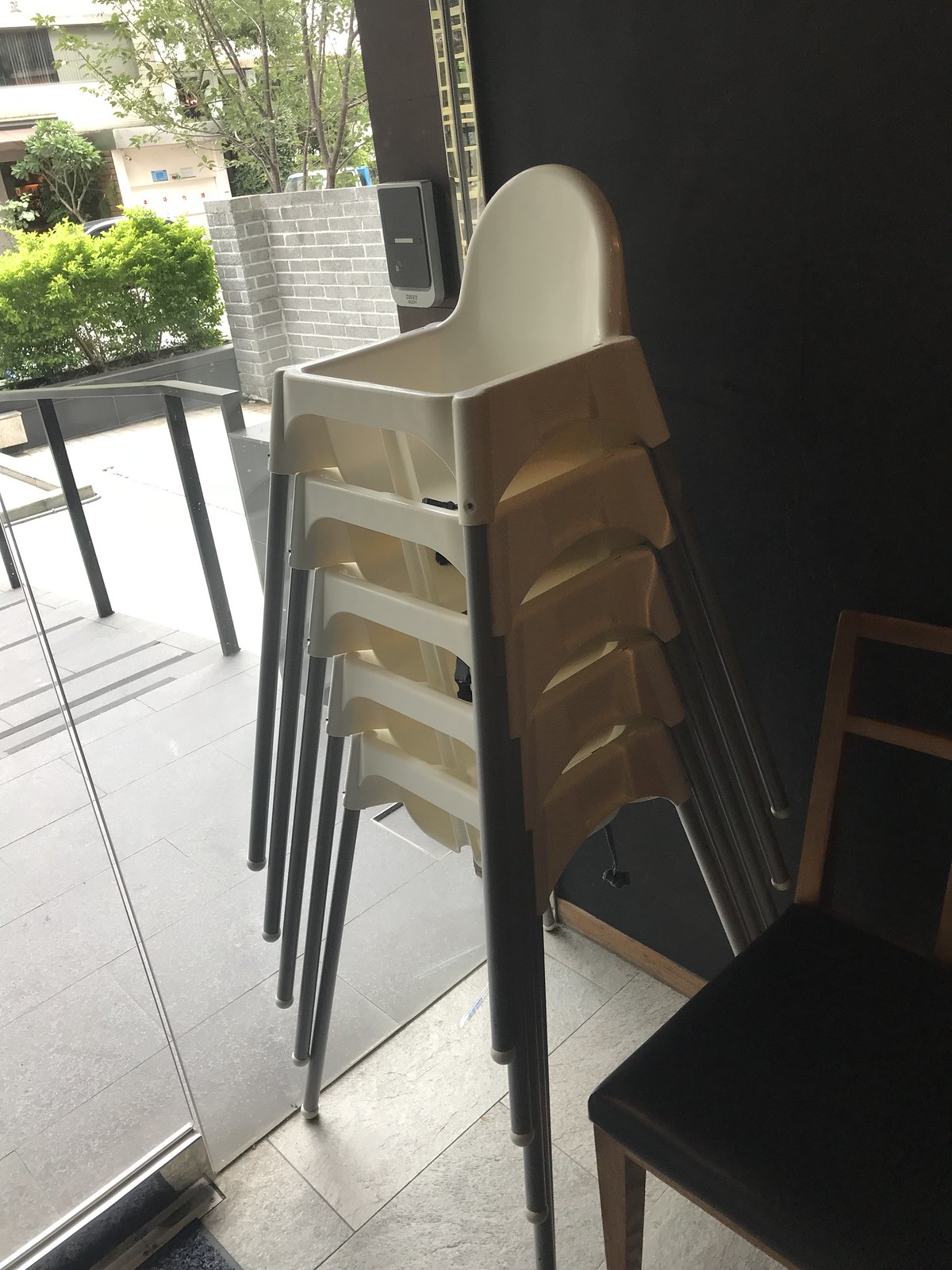The image depicts a stack of five contemporary, cream-colored plastic high chairs, vividly showcasing their design, which includes leg support areas suitable for small children. These chairs are neatly stacked in the corner of a room with dark walls and glass doors that open to an outdoor patio. Beside the stack, a single black chair or stool with a wooden back and darker color padding is visible, adding contrast to the arrangement. The floor inside is tiled in white, providing a clean and modern look. 

Outside the glass doors, an overcast sky casts a shadow on a patio area, which features a brick wall and nearby stairs. The patio is adorned with potted tree plants and a black railing, creating a quaint ambiance possibly used for dining. Across the street, a building, potentially a house, can be seen, suggesting this setting is either a restaurant or café equipped with booster seats for young children, indicated by the multiple small high chairs stacked together.